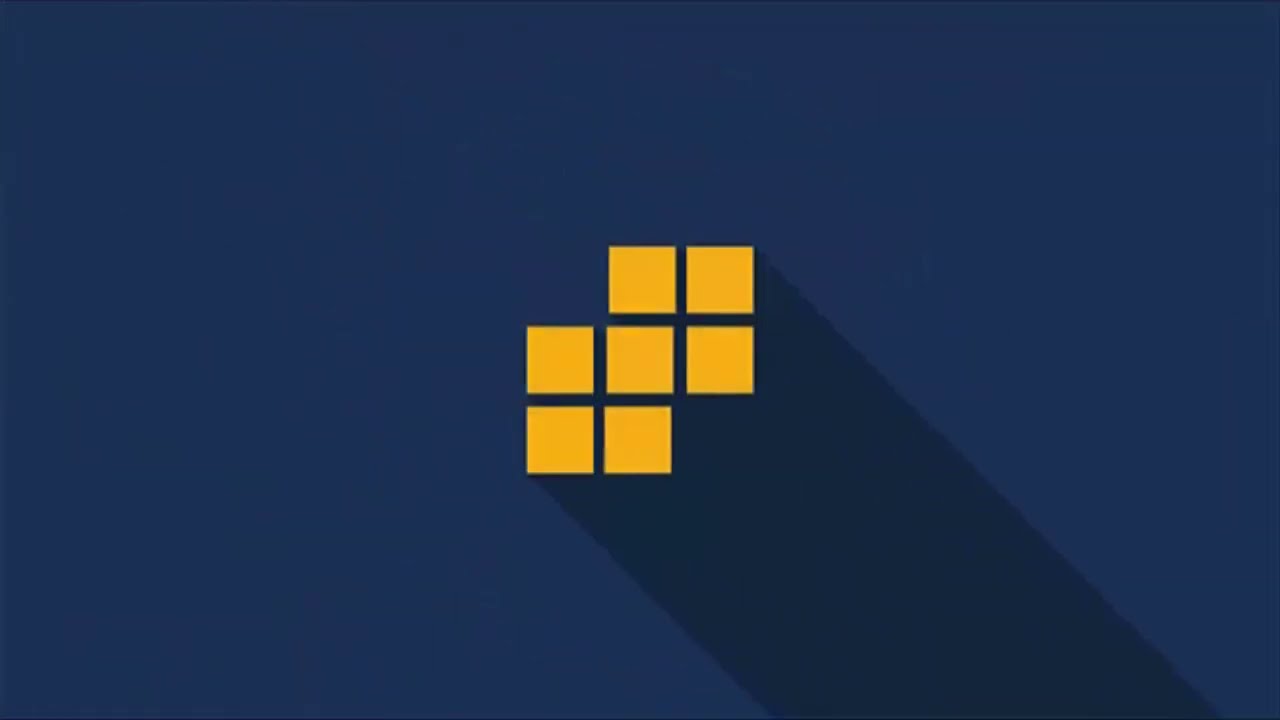The image, likely depicting a logo, features a landscape-oriented graphic with a medium to dark ultramarine blue background. Central to the image is a matrix of seven gold squares (mistakenly referred to as triangles initially), arranged in a formation resembling a three-by-three grid with the top left and bottom right squares missing. The squares form a central horizontal line of three squares flanked by two squares on each side - the left pair aligned at the bottom and the right pair aligned at the top. A dark blue to nearly black diagonal shape extends from the bottom right corner towards the center, adding a shadow-like effect to the design. There is no text or additional elements within the image, giving it a sleek and minimalistic appearance.